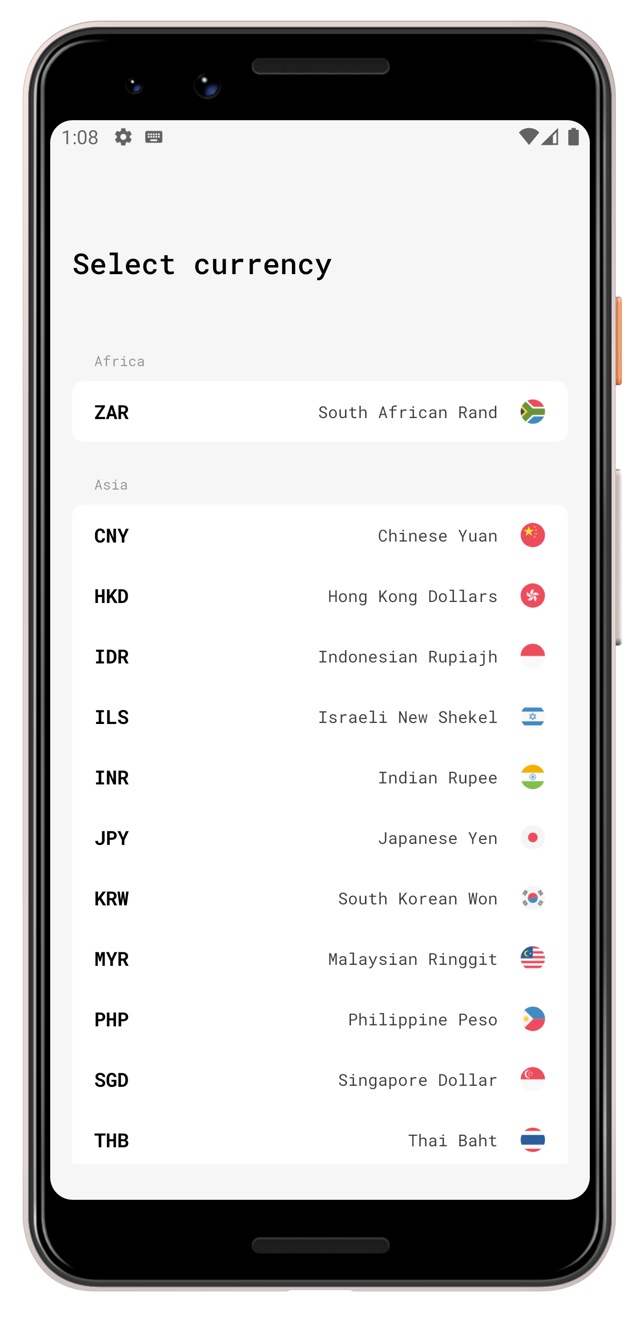In the image, a smartphone is displayed against a completely white background. On the phone's screen, the time reads 1:08 as shown in the upper left corner. Adjacent to the time display, there's a gear symbol indicative of settings, and a keyboard icon is visible as well. On the right side of the screen, status icons for Wi-Fi, signal strength, and battery level are neatly aligned. 

Prominently on the left side of the screen, there's a heading that reads "Select Currency." Below it, the text "Africa, ZAR, South African Rand" is visible at the top of a list. This is followed by another section titled "Asia," listing several currencies along with their abbreviations: "CNY, Chinese Yuan," "HKD, Hong Kong Dollars," "IDR, Indonesian Rupiah," "ILS, Israeli New Shekel," "INR, Indian Rupee," "JPY, Japanese Yen," "KRW, South Korean Won," "MYR, Malaysian Ringgit," "PHP, Philippine Peso," "SGD, Singapore Dollar," and finally "THB, Thai Baht." The corresponding flags of each country are displayed down the right side of the phone screen, enhancing the visual clarity of the currency options.